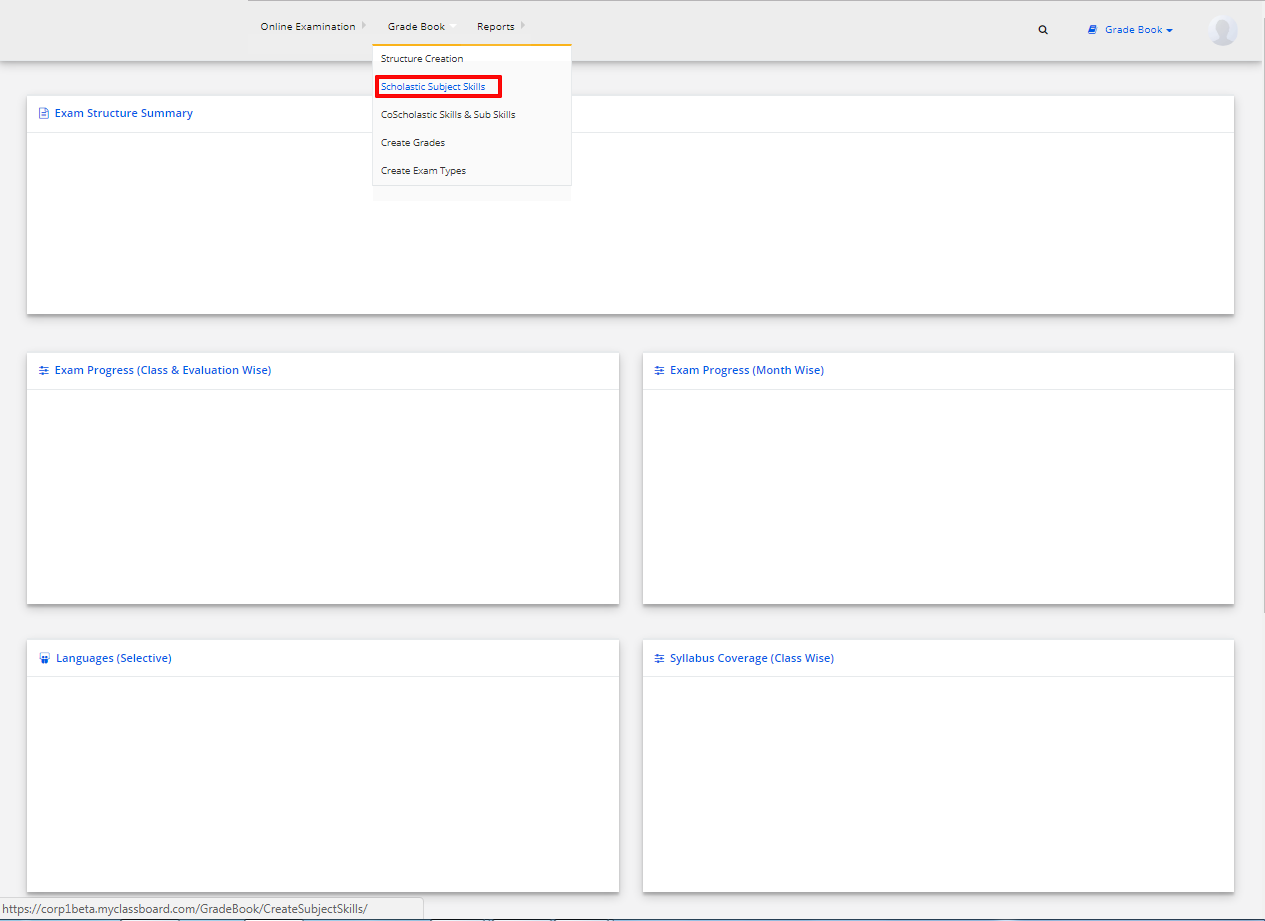This image is a screenshot of a website, presented in a relatively small size which makes the text challenging to read. At the top of the website, there's a grey header featuring several navigation options in black text: "Online Examination," "Gradebook," and "Reports." 

On the right side of the header, there's a search icon represented by a magnifying glass, followed by a small blue icon of a book labeled "Gradebook" in blue text. Further right, there's a circular icon containing a grey silhouette of a person, depicting a head and shoulders.

Beneath the header, on the left side, there is a dropdown menu labeled "Structure Creation," followed by another dropdown option titled "Scholastic Subject Skills" encased in a red border. Below these dropdowns is a partially visible phrase related to skills, likely stating something about "skills and subskills." Further down, there's an option labeled "Create Grades," but the remaining text is too pixelated to read accurately.

In the main content area of the site, there's a large white box with a blue header reading "Exam Structure Summary." This box is empty, except for a horizontal line underneath the header, spanning its entire width.

Below the main box, there are four smaller white boxes aligned in a grid. The first box on the top left reads "Exam Progress (Class and Evaluation Wise)" in blue text, with an empty space below it. To its right, the second box is labeled "Exam Progress (Month Wise)," also empty. 

Below on the left side, the third box is titled "Languages (Selective)" in blue text, with the box content itself being empty. The fourth and final box on the bottom right is titled "Syllabus Coverage (Class Wise)" in blue text, also an empty space.

The website's background is grey, contrasting with the white boxes, and a partially illegible URL is visible at the bottom of the screenshot.